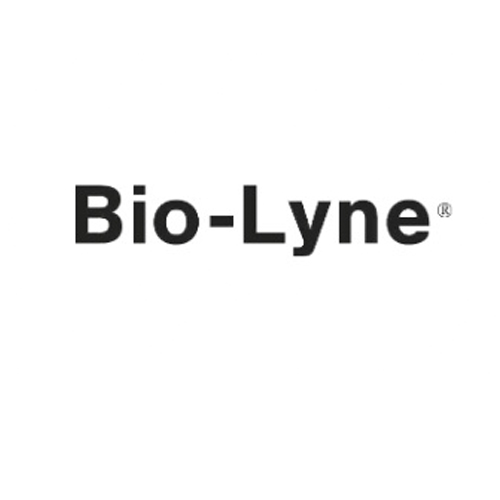The image features a simple design consisting of the company name "BioLyne" in blocky black text, centered on a white background. The name is written with a capital 'B' followed by lowercase 'i' and 'o', then a dash separating it from 'Lyne', which starts with a capital 'L' followed by lowercase 'y', 'n', and 'e'. To the right of the 'e', there is a gray trademark symbol (an 'R' encased in a circle), indicating that the name is a registered trademark. The text appears slightly fuzzy around the edges, suggesting some digital artifacting. The overall design is crisp with the pure white background providing stark contrast to the black letters, drawing clear attention to the company name and trademark symbol.